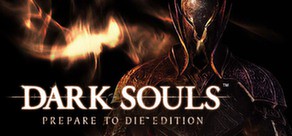The image is a small digital banner advertisement with a predominantly dark, black background illuminated by orange fire-like colors. In the foreground, the central figure is a knight, whose face is obscured by a metal hood and metallic armor covers the chest. The light from the background casts illuminated shades on the knight's armor. Prominently displayed in large white letters across the image is the title "Dark Souls." Beneath this, in smaller white text, it reads "Prepare to Die Edition." There are no additional elements or text on the image.